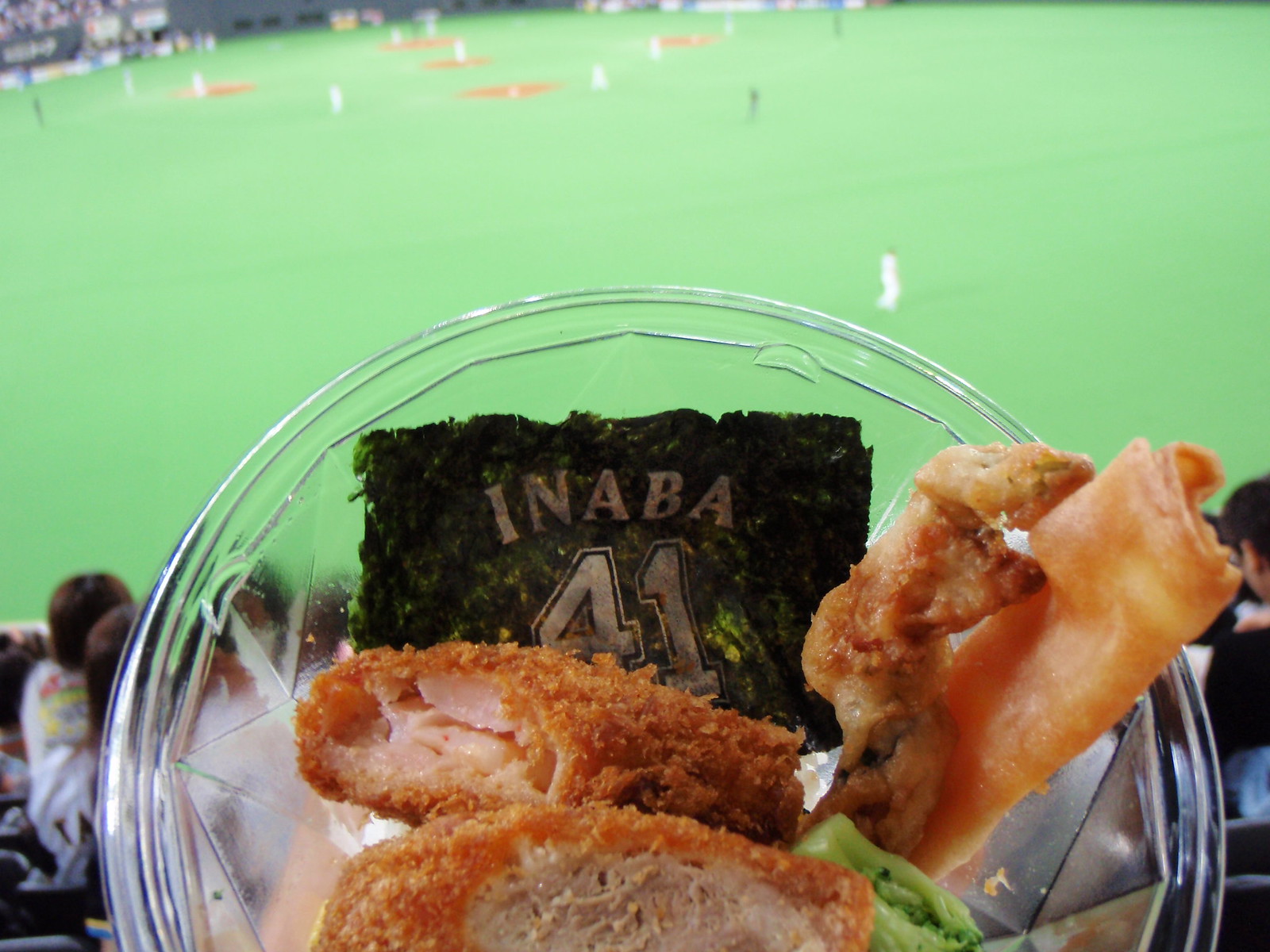A vibrant plate of Japanese ballpark fare is captured in this photo, most likely taken during a baseball game. The clear plastic container, prominently displaying "Inaba 41" on a sheet of nori (seaweed), honors a player from the Occult Swallows team. Featured front and center is a portion of katsu—crispy, breaded meat—sliced open to reveal its tender interior, though the specific type of meat remains indistinguishable. To the right, a small piece of broccoli nestles next to an ambiguous type of fried dough or egg roll. Additionally, a skewer of flavorful yakitori introduces another savory dimension to the array. In the blurred background, the faint outline of a baseball diamond and the green expanse of the field set the scene, enhancing the sensory experience of enjoying a traditional Japanese meal amidst the thrill of the game.